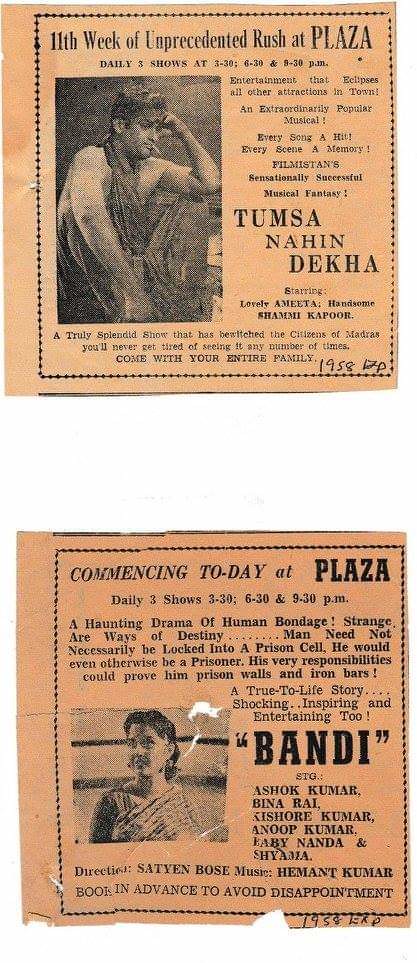This image features two aged newspaper clippings, both with a light brownish or pinky creamy background, indicative of wear and age. The top clipping is bordered with a dashed black line and showcases a black-and-white photograph of a young man sitting with a cigarette hanging from his mouth, leaning his left elbow on his knee and resting his head on his hand, his right arm relaxed by his side. Above him, text reads "11th week of unprecedented rush at Plaza," followed by the showtimes: "Daily shows at 1.30, 4.30, 9.30 p.m." To the right of the photograph, the text "Tumsa Nahin Dekha" is prominently displayed, with additional, smaller text beneath it. Handwritten in the lower right corner is "1958."

The lower clipping, also unevenly cut, announces "Commencing today at Plaza" with showtimes listed as "Daily three shows, 3.30, 6.30, and 9.30 p.m." It features a black-and-white square photograph of a smiling woman in a sleeveless top set to the left side. To the right of the image is the text "Bandi" in quotes, followed by names of characters or actors. This clipping, too, has "1958" inscribed by hand in the lower right corner. Both clippings reflect an older era, with faded, low-quality images and text, offering a nostalgic glimpse into past cinema promotions.